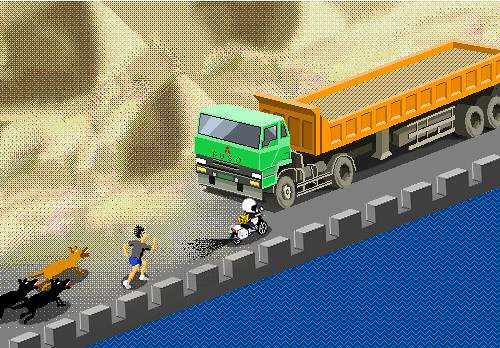This vibrant graphic artwork is presented in a square format. On the bottom left corner, there are three dogs; two of them are black and the one at the front is brown. A person, seemingly moving to the right, leads the dogs. This individual has black hair and is dressed in a grey t-shirt, blue shorts, and white shoes. Positioned ahead of this person is a white motorcycle, ridden by another individual. The motorcycle rider is adorned with a white helmet and a yellow backpack. Dominating the scene on the opposite side of the road is a long, large truck. Unfortunately, the truck's front section is not fully visible in the image. This dynamic composition captures a bustling moment filled with movement and vibrant details.